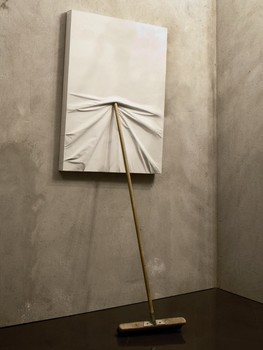The image depicts a seemingly empty art exhibit with a minimalist setup. The centerpiece is an intriguing installation featuring a blank white canvas mounted on a beige-brown, shadowy wall, with sections of the wall revealing gray and concrete-like textures near the right corner. The floor is dark, resembling a deep wooden finish. The main focus is a long wooden broom with black bristles, propped at an angle against the canvas. The broom handle appears to be wedged into the middle of the canvas, creating an illusion that the canvas is being "eaten" or held up by the broom, with the handle forming a mouth-like effect. This interaction causes the canvas to wrinkle and distort at the point of contact and below, while the upper part remains smooth and flat. The setup, seemingly staged, evokes a potential metaphor about the supportive and often underrated role of blue-collar work in sustaining artistic endeavors. The entire scene is rendered in shades of brown and white, devoid of other colors, enhancing its stark, conceptual nature.